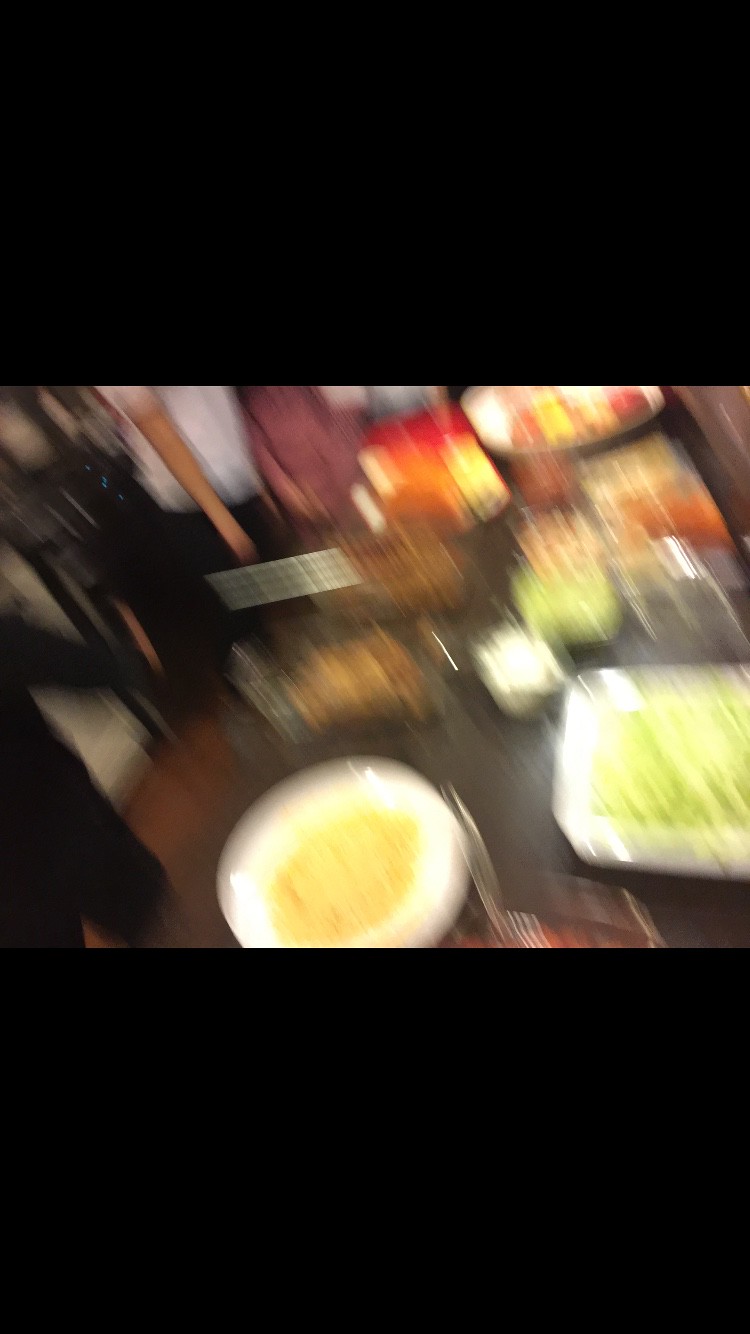The central feature of this image is a blurry, horizontally-oriented photograph of a long table laden with various dishes, set against a vertical black background. The table, likely brown, is cluttered with an assortment of food that is difficult to identify due to the blurriness. To the bottom left, a round bowl appears to hold a yellow substance, while on the bottom right, a square bowl seems to contain chopped green lettuce. Additional indistinct dishes populate the table, potentially including pasta, salad, chicken, and fruit. The image, likely taken during a meal either at a restaurant or a large gathering, shows smudged figures in the background. A man in a white short-sleeve shirt tucked into black pants and a woman in what seems to be a pink dress are faintly visible. The photo suffers from motion blur, suggesting the camera was moved accidentally while capturing the scene. The peculiar aspect ratio, with black bars cropping the top and bottom, hints at a horizontal picture viewed in portrait mode.